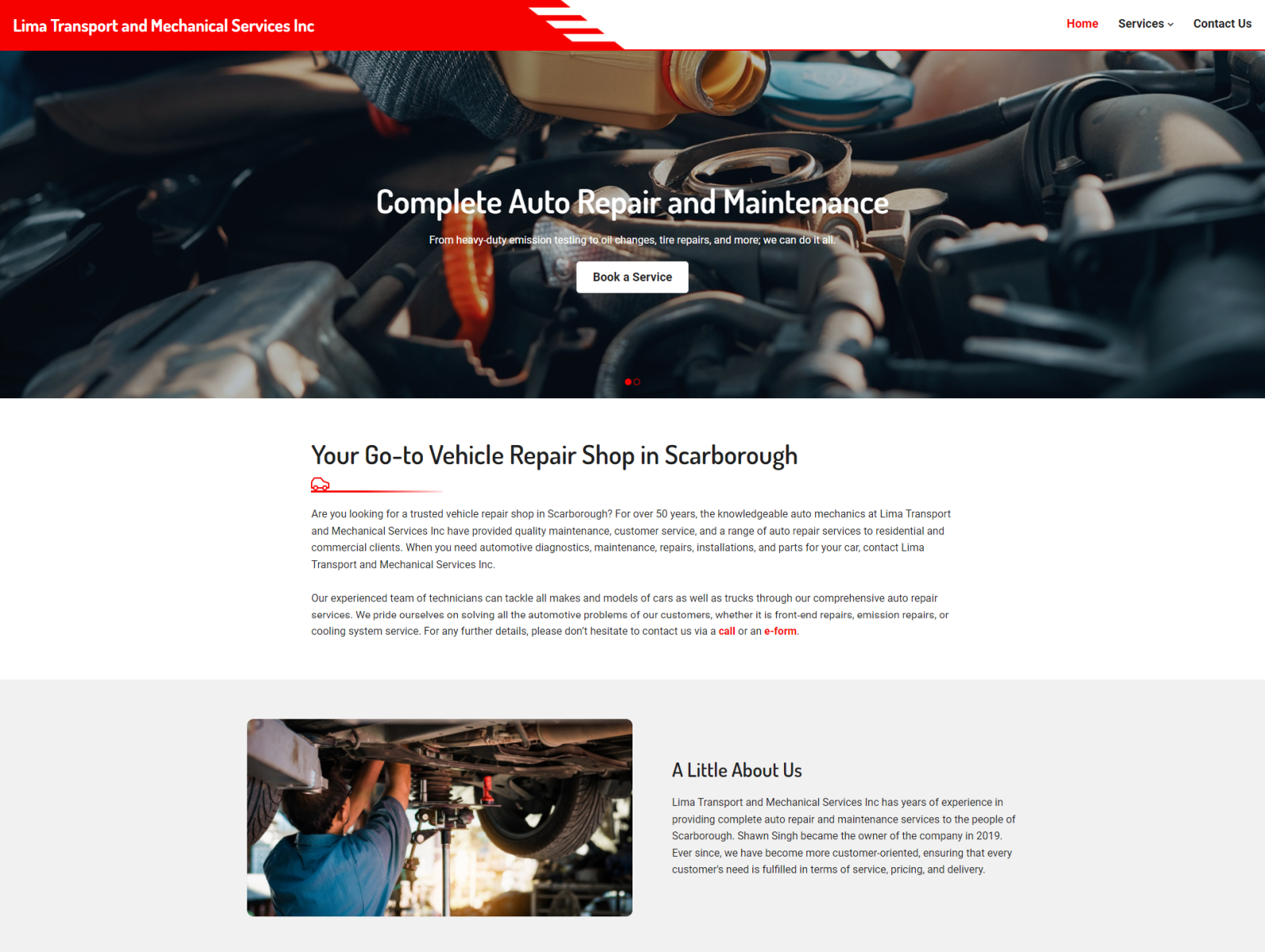The image is a detailed screenshot of a business webpage related to automotive services. At the center, prominently displayed against a background showing the inner components of a car engine with a person adding oil or another fluid, is the title: "Complete Auto Repair and Maintenance." The text below the title reads: "From heavy-duty emission testing to oil changes, tire repairs and more, we can do it all." There is also a call-to-action button that says, "Book a Service.”

In the upper left corner, within a red rectangle, it reads, "Lima Transport and Mechanical Services." Directly beneath this title, the subheading states, "Your go-to vehicle repair shop in Scarborough." Unfortunately, the text below this subheading is too small to be legible.

Below that section is an image of a mechanic dressed in a blue short-sleeve shirt. The mechanic is standing under a car—presumably elevated on a hydraulic lift—focused on repairing its undercarriage. A car wheel is visible to the image's right.

To the right of the mechanic’s image, there is a section titled "A Little About Us," accompanied by a paragraph describing the business, which is too small to read in detail. This screenshot effectively summarizes the services and credibility of the complete auto repair and maintenance shop.